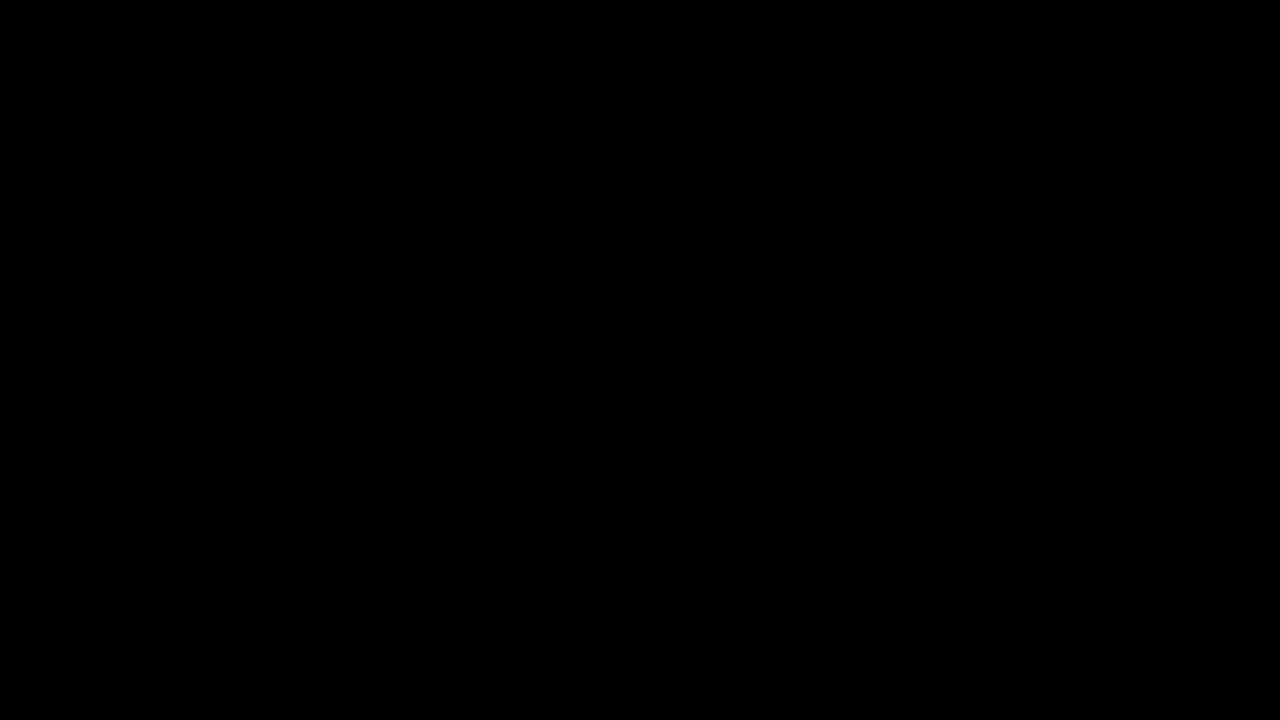This image depicts a large, completely black rectangle displayed on a computer screen. The rectangle spans approximately 7 to 8 inches in width and about 5 inches in height, fully filled in with an intense, dark black color without any text, numbers, or borders. The blackness is as profound as that of a dark room or a locked closet, exuding a sense of total visual absence, similar to the momentary blindness caused by a flashbulb. The image is uniformly black throughout, with no variations or white spots, giving the impression of either a simplistic artistic backdrop or perhaps an abstract representation akin to a black hole. It's a stark, featureless, and infinite black space, leaving much to the viewer's imagination.